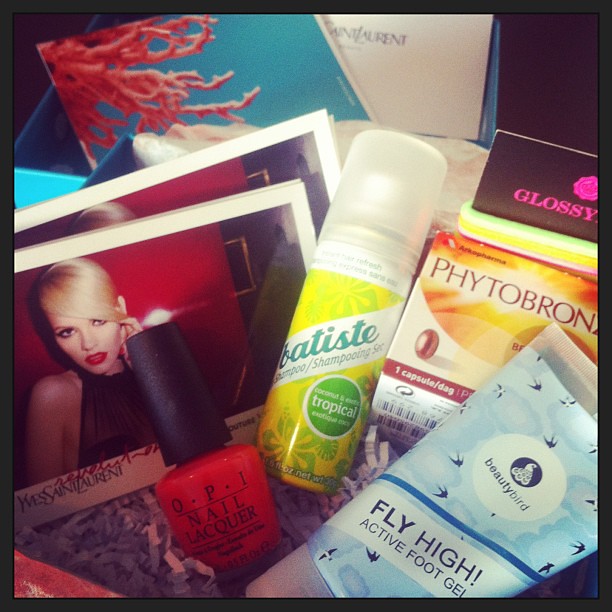This image depicts an intricately packed makeup subscription box, filled with various beauty items and detailed promotional materials. At the top left, a postcard rests inside a blue box, adorned with coral reef illustrations in red. Beside it, there's an envelope branded with "Yves Saint Laurent" in black lettering. Another blue box below it contains photographs of a young blonde woman with striking red lipstick, heavy black mascara, and a black shirt with cutouts, set against a red backdrop.

The main compartment of the box is cushioned with purple shredded paper, providing a bed for the featured products. Central to the display is a yellow bottle of Batiste dry shampoo, decorated with green flowers and marked with "Tropical Scent" inside a green circle. Adjacent is a distinct glass bottle of OPI nail lacquer, striking in red with "OPI" and "nail lacquer" inscribed in black, paired with a tall, black plastic cap. Nearby, a tube labeled "Beauty Bird Fly High Active Foot Gel" in a blue tone stands out, while a small box, labeled "Phyto Bronze One Capsule," is tucked behind. These elements, harmoniously arranged, present an enticing array of beauty essentials against the textured backdrop of shredded paper.